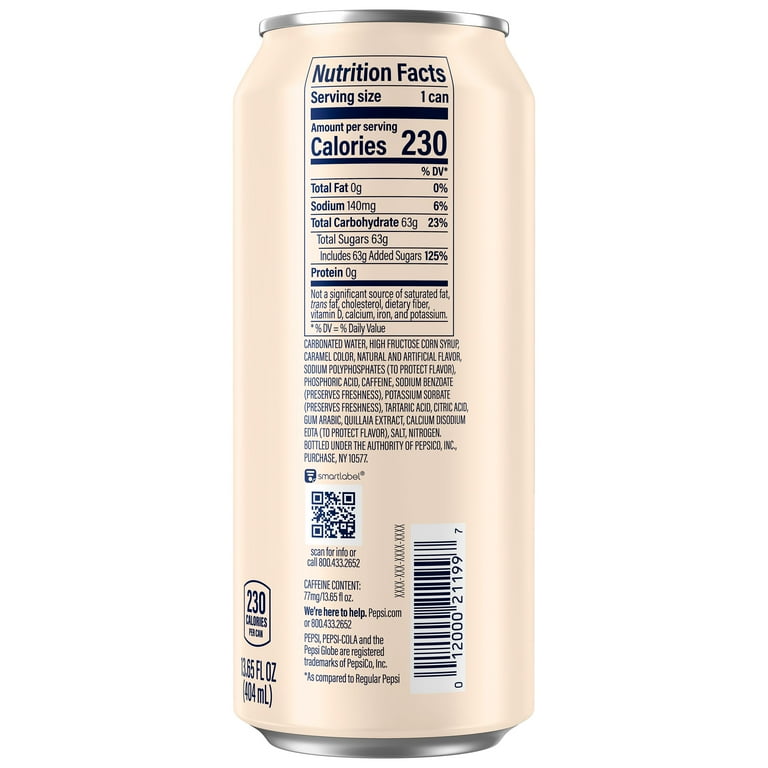The image depicts the back of a taller-than-wide, beige or cream-colored aluminum can of Pepsi, providing detailed nutritional information and listing various ingredients. The text on the can notes that it contains 230 calories, 0 grams of protein, 63 grams of total carbohydrates, 63 grams of sugar, and 140 milligrams of sodium per serving. Ingredients include carbonated water, high fructose corn syrup, caramel color, and various other additives and preservatives. Additionally, there's a QR code for more information, a barcode for scanning at purchase, and Pepsi branding including customer service contact details and caffeine content. The top of the can is silver, and the detailed nutritional facts and ingredients list are prominently visible, affirming that the drink is a Pepsi product.